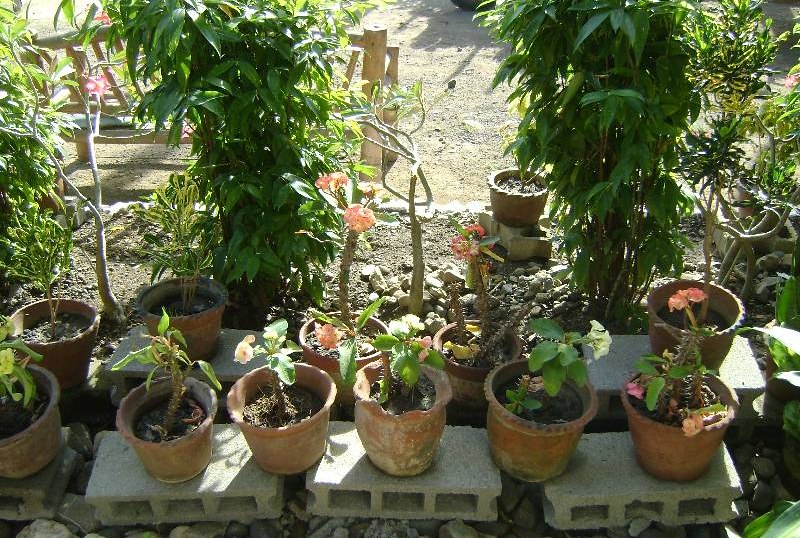The photograph showcases a serene garden scene in a yard. In the foreground, a series of gray cinder blocks, each with hollow square sections, are meticulously laid on their sides, forming a base for two neat rows of orange terracotta pots. These pots contain an assortment of plants, some bearing vibrant flowers in shades of pink, orange, and white, while others have lush green foliage. Toward the background, a wooden bench, possibly made from light brown wood, sits invitingly amidst a large expanse of light brown dirt, accented with small rocks. Surrounding the area, larger plants and small trees rise prominently, their long brown stems crowned with either dark or light green leaves. The sunlight filters through these taller plants, casting a gentle glow on the terracotta pots. Additionally, the scene includes glimpses of a grey soil walkway and a wooden fence peeking at the top of the image.